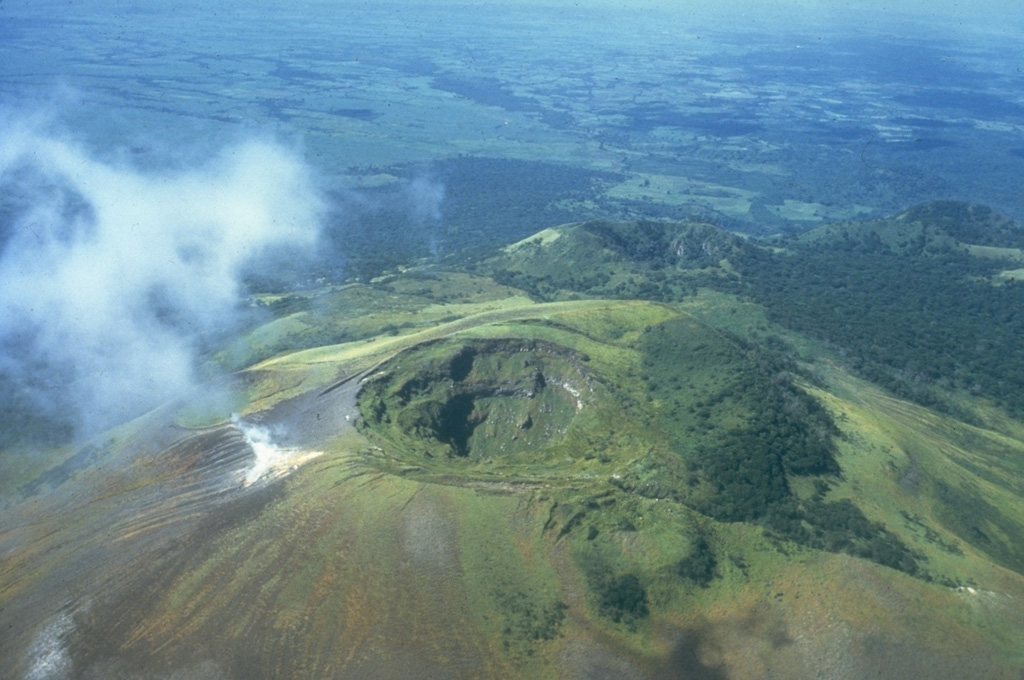The aerial image captures a verdant landscape characterized by a distinct crater-like depression in the center of a hill, reminiscent of a small volcano with a central hole leading downward. The scene, observed from above, possibly taken from an airplane or drone, reveals a rich tapestry of greens with varying shades, indicating dense vegetation and trees that extend into the distance. Around the crater, one can see grass lining its edges, adding to the lush feeling of the landscape. Above the crater, clouds meander, initially giving the illusion of smoke. The terrain in the background flattens out, stretching far into the horizon, where the greenery transitions into a more muted, bluish hue due to the distance. The sky is absent from the frame, focusing the viewer's attention solely on the detailed and expansive natural scenery below.